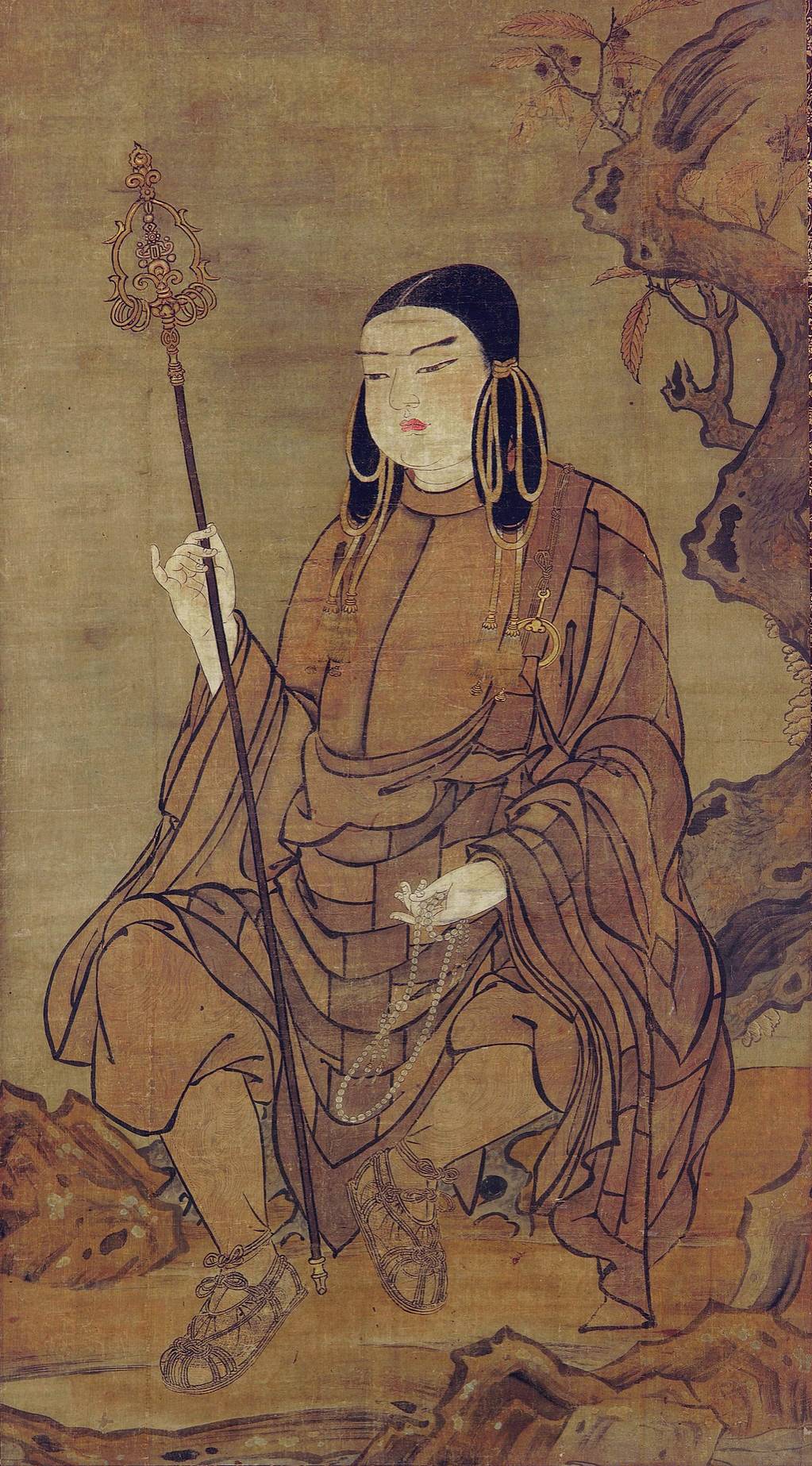In the image, there is a detailed depiction of an ancient Asian woman, likely influenced by traditional Chinese or Japanese artistry. She has black hair, styled into two buns on the side of her face, with ropes tied around them. The woman is seated, possibly on a tree stump, amidst a natural setting that features trees and rocky, brown ground. She wears an elaborate brown tunic adorned with heavy ropes and beads, giving her an appearance reminiscent of a Buddhist or Shinto practitioner.

In her right hand, she holds a long black staff, akin to a scepter, while her left hand appears to be pinching her ear. Additionally, she seems to have some jewelry, possibly a necklace, in her grasp. Her attire includes open-toed sandals with multiple buckles. The overall ambiance suggests she might be engaged in meditation or prayer, potentially warding off evil spirits, surrounded by an ancient, tranquil environment.